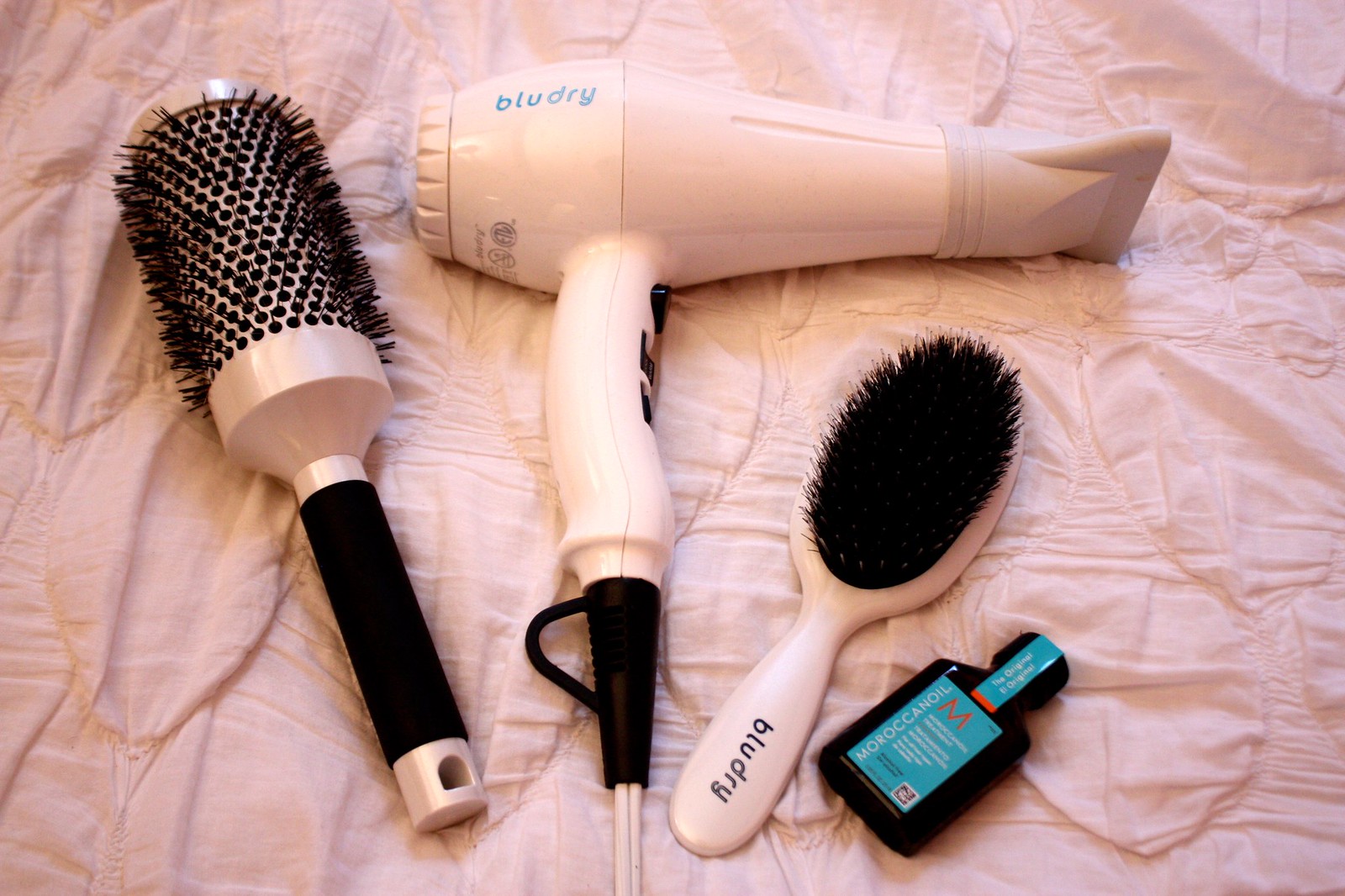This photograph captures an array of hairstyling tools meticulously arranged on a pink comforter. The tools, featuring matching pink tones that complement the fabric, include a variety of essential items for hair care. To the left, there is a pink round brush with thin black bristles and a black handle that includes a hole for hanging. Accompanying this brush is a pink hair dryer branded with "BLUDRY" on its side. This dryer features a black-grip section where the cord attaches and a flat end. Adjacent to the hair dryer, a flat, oblong brush branded with "BLUDRY" and equipped with black bristles is positioned. Finally, completing the ensemble is a small black bottle of Moroccan Oil, identifiable by its blue label and distinctive orange "M."